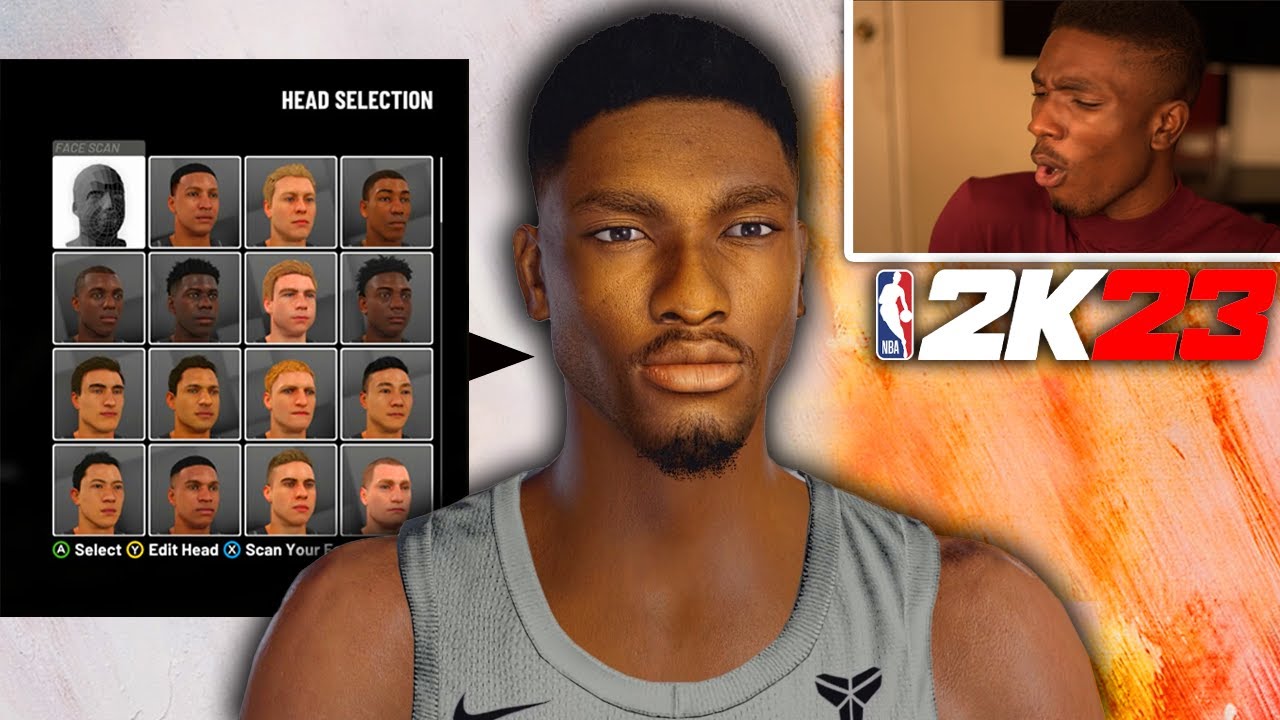In this detailed preview of the NBA2K23 game, we see a character model of a player wearing a gray jersey. Prominently displayed on the left side of the jersey is a black Nike logo, while on the right side is a unique three-triangle black logo with small gaps between the connections. The player, a black male, is standing in the center of the screen, staring straight ahead. His hair is styled with longer hair on top and shaved sides, paired with a mustache and whiskers on his chin.

In the upper right-hand corner, there is a smaller box featuring a live reaction of the actual individual whose face has been scanned into the game. He is wearing a maroon t-shirt and looking to the side with a shocked expression, his mouth open in disbelief. Below this box is the NBA logo and the 2K23 logo, with "2K" in white and "23" in red, set against a background of a tan and red wood basketball court.

Additionally, on the left-hand side of the image, there is a selection box labeled "Head Selection" in white capital letters against a black background. It displays four rows of four headshots each. The top-left headshot has a white background with a gray head and the label "Face Scan," while the remaining headshots feature various faces with gray backgrounds. At the bottom of this selection screen, there are three options: a green circle "A" for Select, a yellow circle "Y" for Edit Head, and a blue circle "X" for Scan Your Face.